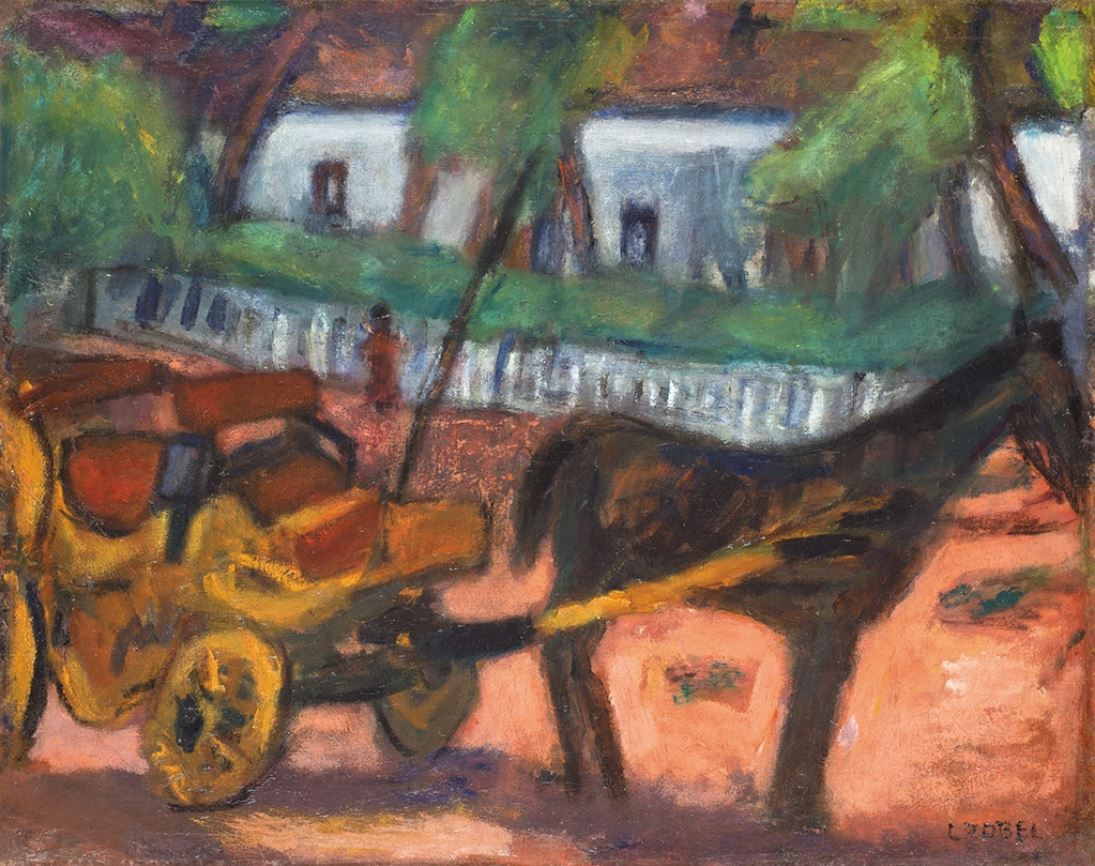The image depicts a post-impressionist painting characterized by its abstract and fragmented style, likely created with watercolors. Dominating the foreground on the right is a dark brown horse or donkey, its nose extending off the canvas, and it is harnessed to a vibrant yellow carriage with red seats. The carriage, notable for its brightness, anchors the composition. In the middle distance, a man wearing a black hat stands outside a white house surrounded by trees and greenery, perhaps a yard or garden. This house is part of a cluster of buildings featuring whitewashed walls, hinting at a serene rural setting. The ground is painted in earthy hues of orange and brown, enhancing the warm, natural feel of the scene. A signature, partly legible as "L-something-bell," is inscribed in the bottom right corner, further authenticating the artwork.